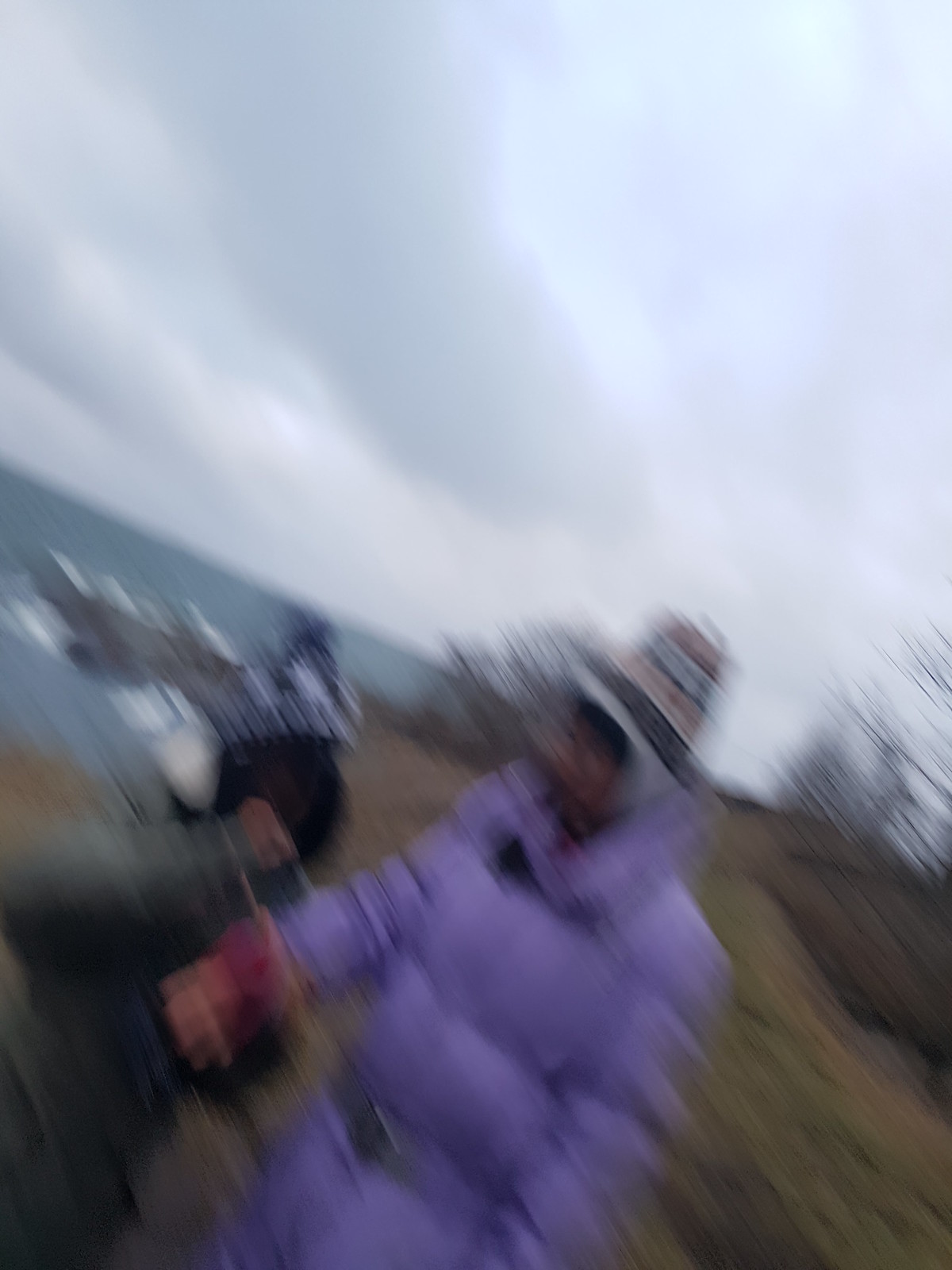This rectangular photograph, taken during the day in a mountainous hilly area, is exceptionally blurry, seemingly captured with a rapidly moved lens. Despite the lack of clarity, several elements are discernible. A somewhat discernible human figure is positioned diagonally from the lower left to the upper right, clad in a light lavender parka and wearing a striped hat. While the person's facial features and gender are indistinguishable, there is a hint of dark hair visible. Behind the figure, a vague form appears, possibly another person or an object, characterized by a dark black base and a gray top. The background features a diagonal skyline that meets the horizon over what seems to be a green or mountainous landscape. The sky has an abstract, swirling pattern in shades of gray, black, and white. On the right side of the image, the silhouettes of trees add to the overall indistinct and chaotic composition of the photograph.